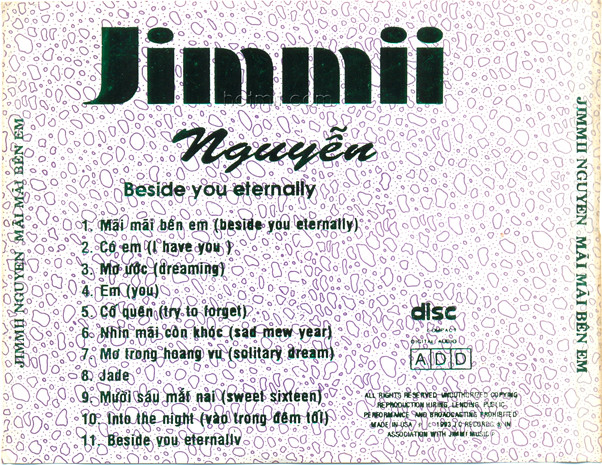This square image showcases the front cover of a worn CD case with an animal print background in shades of white and gray. Prominently displayed at the top in large black letters is the artist's name: "JIMMII." Below that, in cursive, it reads "win," followed by "NGUYEN" in black letters. The album title, "Beside You Eternally," is also featured beneath the artist's name. The cover lists 11 songs in another language, with English translations provided in parentheses. The song titles include "My My Ben M (Beside You Eternally)," "Ko M (I Have You)," "Mo Your Duck (Dreaming)," "M (You)," "Ko Kien (Try to Forget)," "Sad New Year," "Solitary Dream," "Jade," "Sweet Sixteen," "Into the Night," and a repetition of "Beside You Eternally." Vertically written on the sides of the CD is "Jimmy, Win, May, May, Ben, M." In the lower right-hand corner, it says "disc," accompanied by smaller, unreadable text. The overall design features a monochromatic color palette with hints of purple, black, tan, gray, and green.